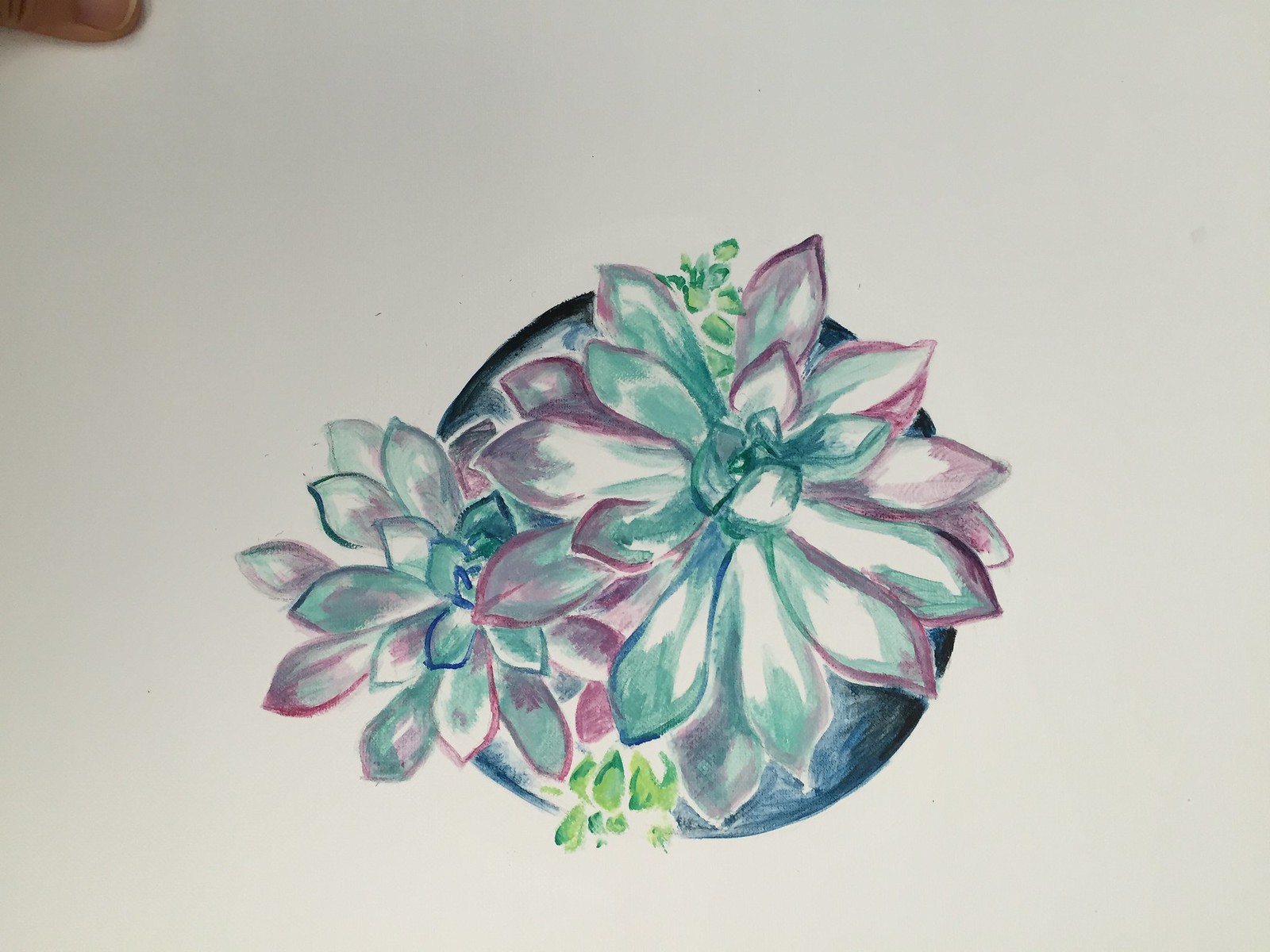This image features a detailed drawing on a white piece of paper. Dominating the center is a blue circle outlined in black. Inside this circle are two meticulously drawn flowers, adorned with green leaves positioned at the top and bottom. The flower on the left is slightly smaller than the one on the right. Each flower showcases a blue center that gradually transitions into pink as it extends outward through three layers of long, skinny petals. The intricate petals culminate in a pink edging. A thumb is visible in the top left corner of the image, adding a human touch to the scene. The bottom leaves also exhibit a mix of green and purple hues, adding depth and texture to the composition.